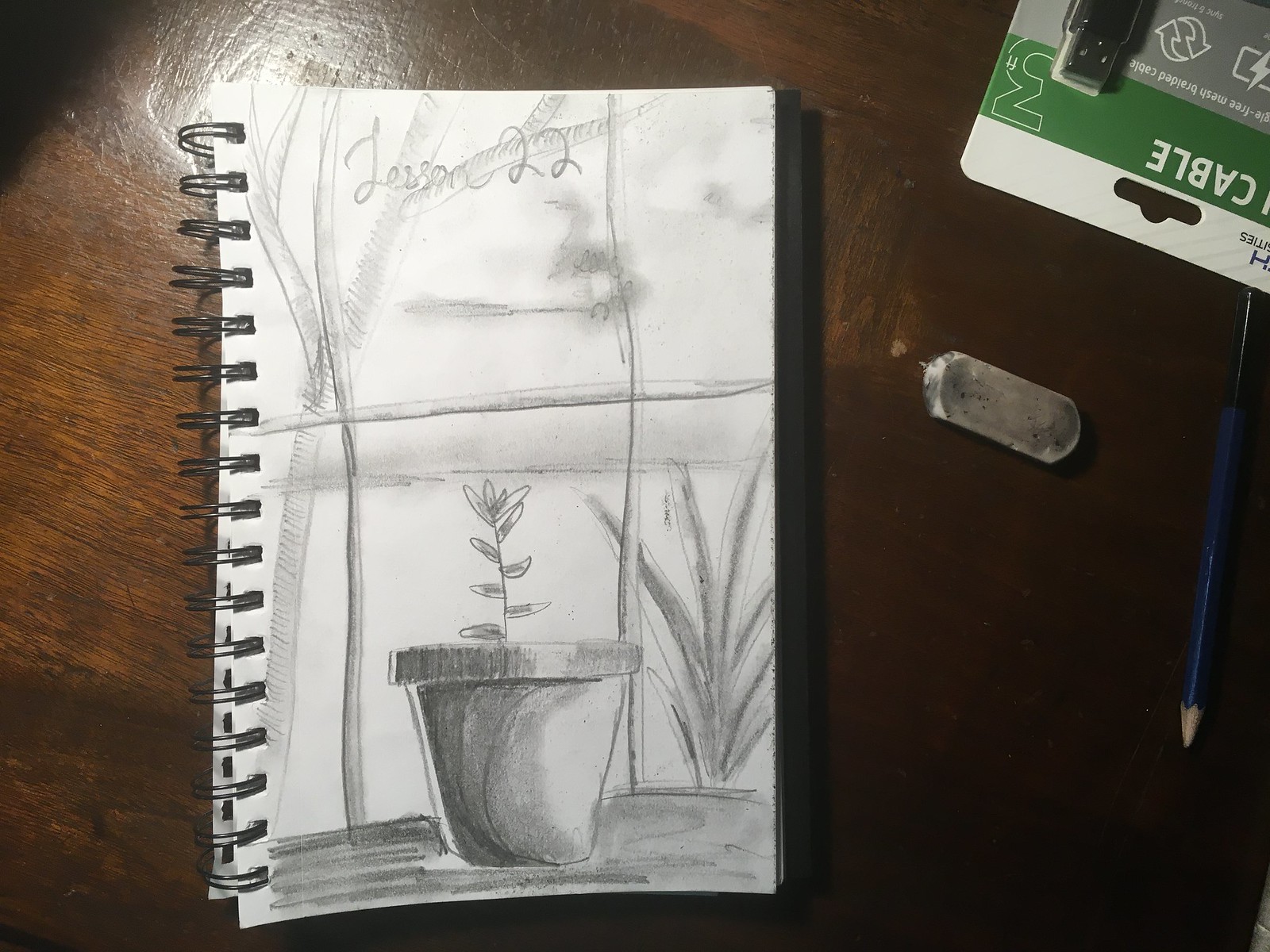The image displays a notebook featuring intricate black and white artwork on a white sheet of paper. The artwork depicts a flower pot with a plant growing out of it, complemented by another plant situated to the right of the pot. The notebook’s black spirals are visible along the left side of the artwork. Positioned to the right of the notebook is a white and black eraser, alongside a blue pencil.